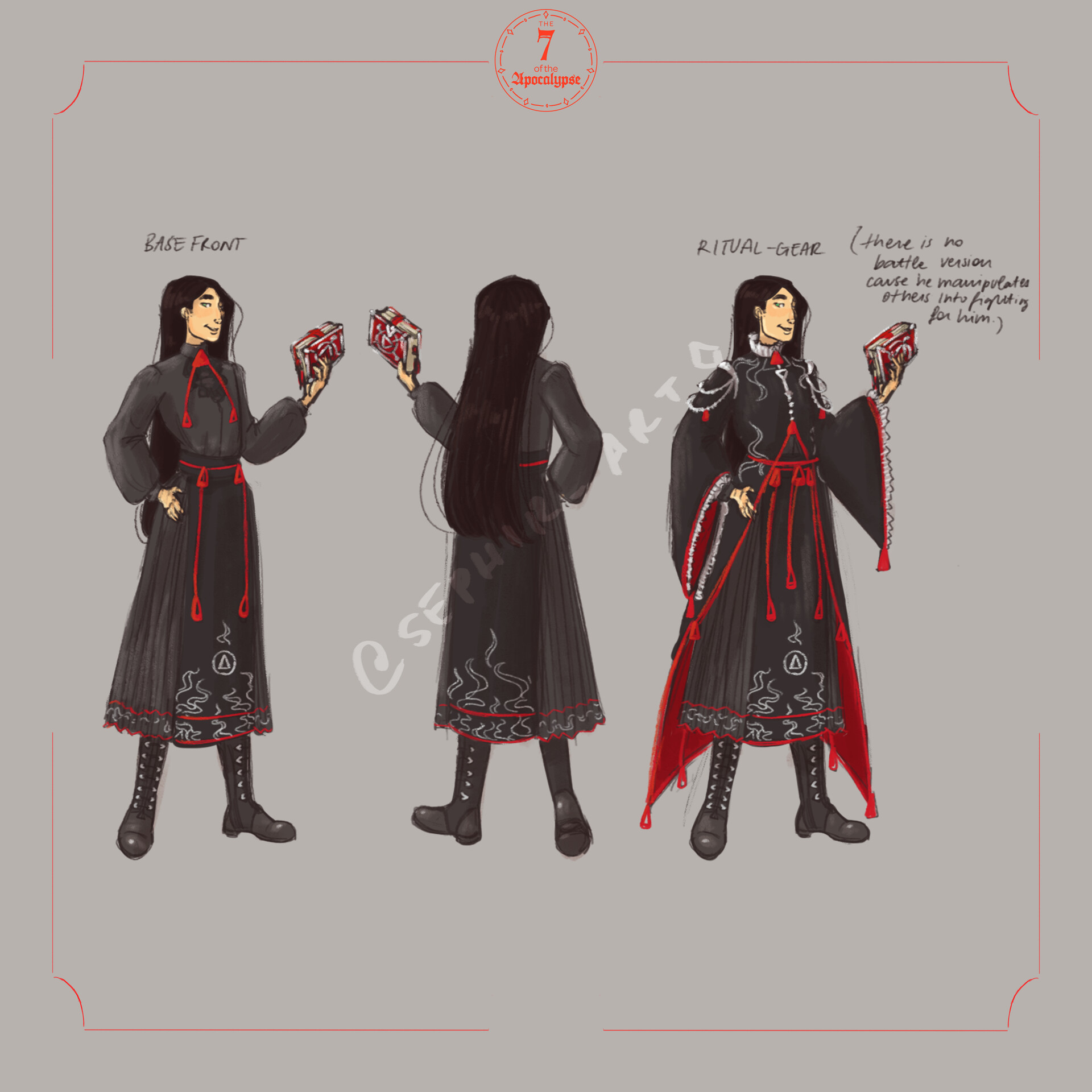The image is a detailed concept drawing of a character, potentially for a story or a game, showcasing both their "base front" and "ritual gear" outfits. The character, who appears ambiguous in gender, is adorned in Asian-inspired traditional attire with black and red as the dominant colors. They have long, straight black hair and wear a sly smirk. The "base front" outfit features a long, black dress-like garment with a red upside-down V at the top and a thin red belt extending downward with two red strips. Complementing this are black boots and a red and white book held in the left hand.

The "ritual gear" is more elaborate, with the garment extending into a cape-like ensemble with long, flowing sleeves. This outfit has more intricate red patterns, especially on the arms and back. The character is again seen holding the red and white book. Notably, a cursive text near the ritual gear mentions, "there is no battle version because he manipulates others into fighting for him," hinting at the character's manipulative nature.

The background of the drawing is gray, adding contrast to the vivid red and black of the character's attire. Additional details include small, hard-to-read black font labeling above the outfits and a social media handle, "@SaphiraArt," presumably credited to the artist.